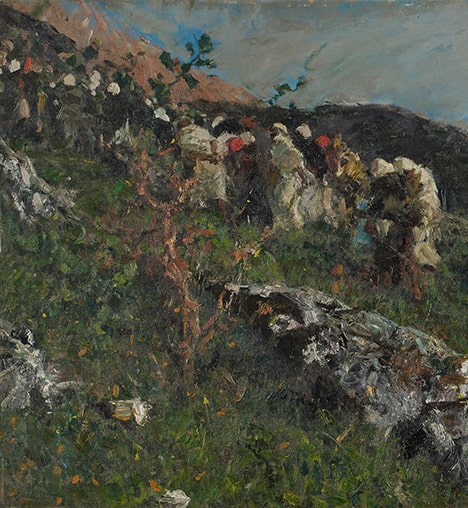The painting is an impressionist outdoor scene that features a muted color palette with dull greens, browns, grays, and occasional patches of blue in the sky. Central to the composition is a line of people, seemingly of African American descent, walking single-file up a steep hillside or mountain. They are dressed in robes and hats, with some garments appearing white and others black. The figures have their backs to the viewer, moving away from a rock outcropping and a prominent, leafless tree that stands stark against the subdued backdrop. Nearby, a fallen tree contributes to the somber atmosphere. The sky is predominantly gray, suggesting an overcast day with faint glimpses of blue. Although the painting employs big shapes and broad brushstrokes, it is meticulously detailed, capturing an evocative moment in a dark, contemplative landscape.